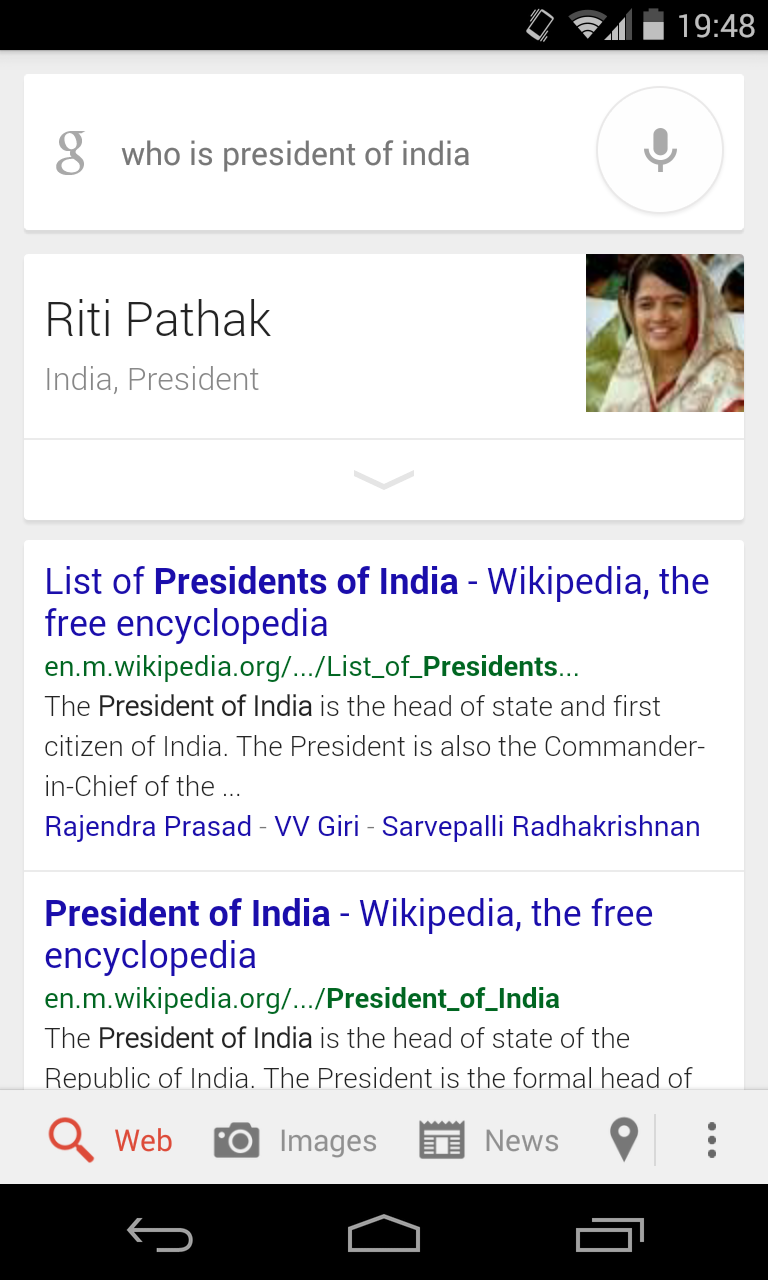The screenshot appears to be from a smartphone, evidenced by the phone icon, Wi-Fi icon, and battery indicator at the top of the screen, which shows 19:48 as the current time. The Google search app is open and a query, "Who is the president of India?" is entered in the search bar. To the right of the search bar is a microphone icon encased in a dark gray circle. The overall background of the page is light gray.

Below the search bar, the first search result displays the text "Riddhi Pathak, India, president" with an accompanying image, likely of the said individual. Adjacent to this result is a drop-down button. Following this result, there are two nearly identical entries linking to Wikipedia, titled "List of Presidents of India - Wikipedia, the free encyclopedia" and "Presidents of India - Wikipedia, the free encyclopedia."

At the bottom of the screen is a navigation bar featuring a red magnifying glass with the label "Web" beside it. Adjacent to this icon, from left to right, are icons and labels for "Images" (a camera icon), "News" (a newspaper icon), and "Map" (a map icon). To the far right are three horizontal dots, indicating additional options.